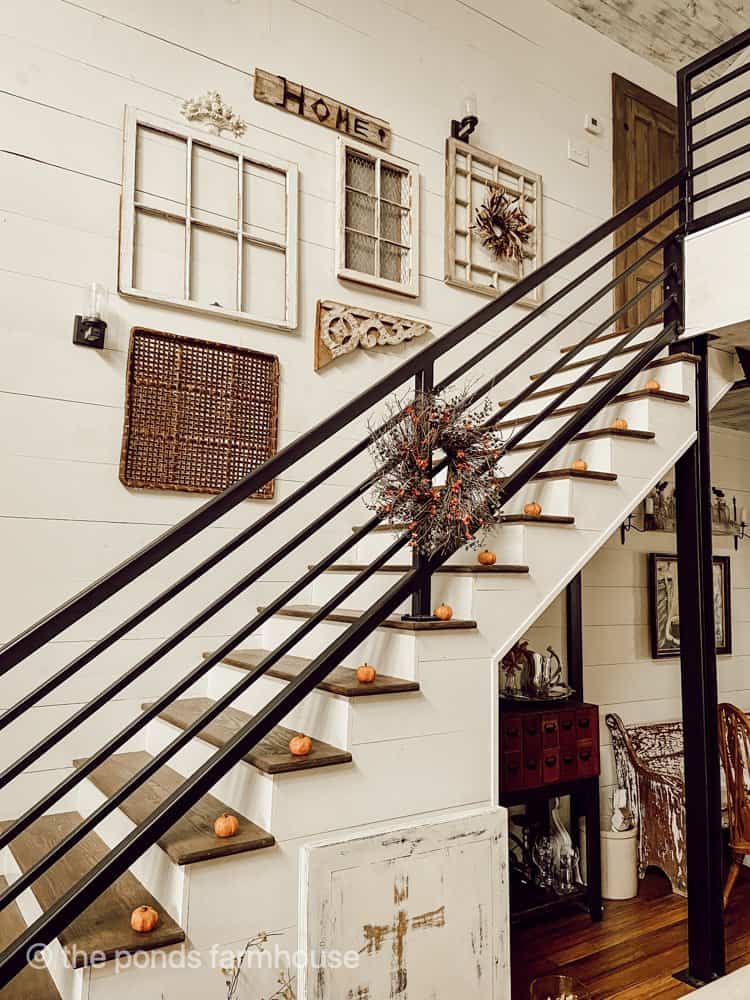The image is a vertically aligned photograph taken inside a predominantly white home, focusing on a stairway that climbs from the lower left to the upper right. The steps feature brown wooden tops with white risers and are bordered by white-painted wooden sides. Black metal railings accompany the staircase, consisting of both thicker top and bottom rails accompanied by four thinner ones. Each step is adorned with small orange pumpkins. The surrounding walls, made of white horizontal wooden slats, are decorated with various items. Pictures are hung along the staircase wall, including a square brown wicker decoration and several white and off-white frames without pictures inside. A sign bearing the word "home" and another board in the lower-left corner inscribed with "The Ponds Farmhouse" are visible. At the top of the stairs, on the upper right, stands a closed brown wooden door next to a wall-mounted thermostat. Downstairs, partially visible in the lower right, the floor is dark wood tile with more pictures hung on the wall and a small area beneath the stairs featuring a cart with teacups and a shabby chic wood bench.